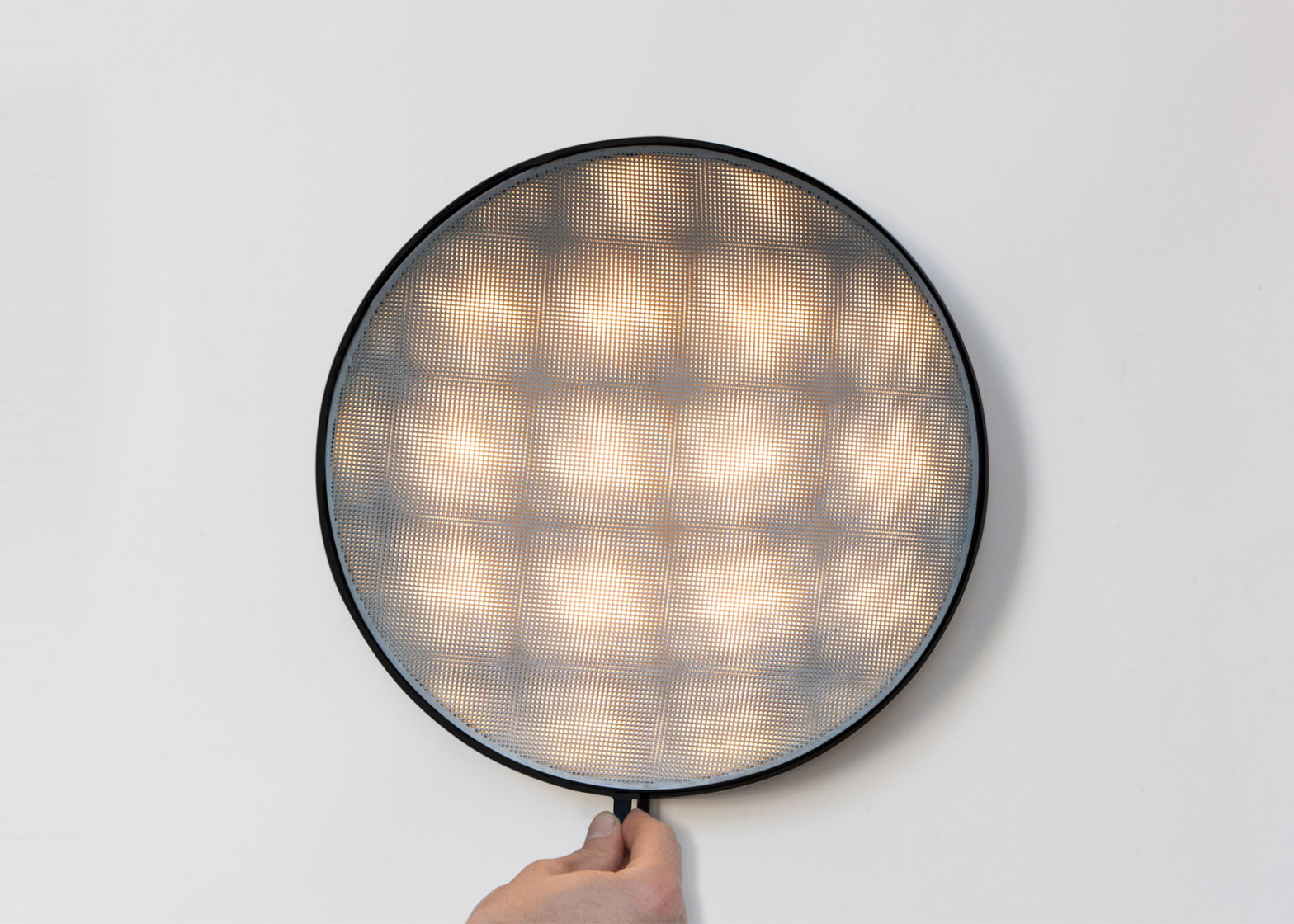In this image, a white hand emerges from the bottom, gripping a handle or stem attached to a large, circular black object, resembling a tennis racket in shape but with notable differences. The circular object features a fabric or screen at its center, patterned with a grid of squares. These squares seem to emit a soft, bright light, giving a luminous appearance with a gradient effect from bright white at the center to the edges. The squares number around 12 or 13 full squares with additional half squares cut off by the circle’s perimeter. The entire composition is set against a light gray or white background, possibly a wall or table surface, and the illumination has a subtle light orangish hue.